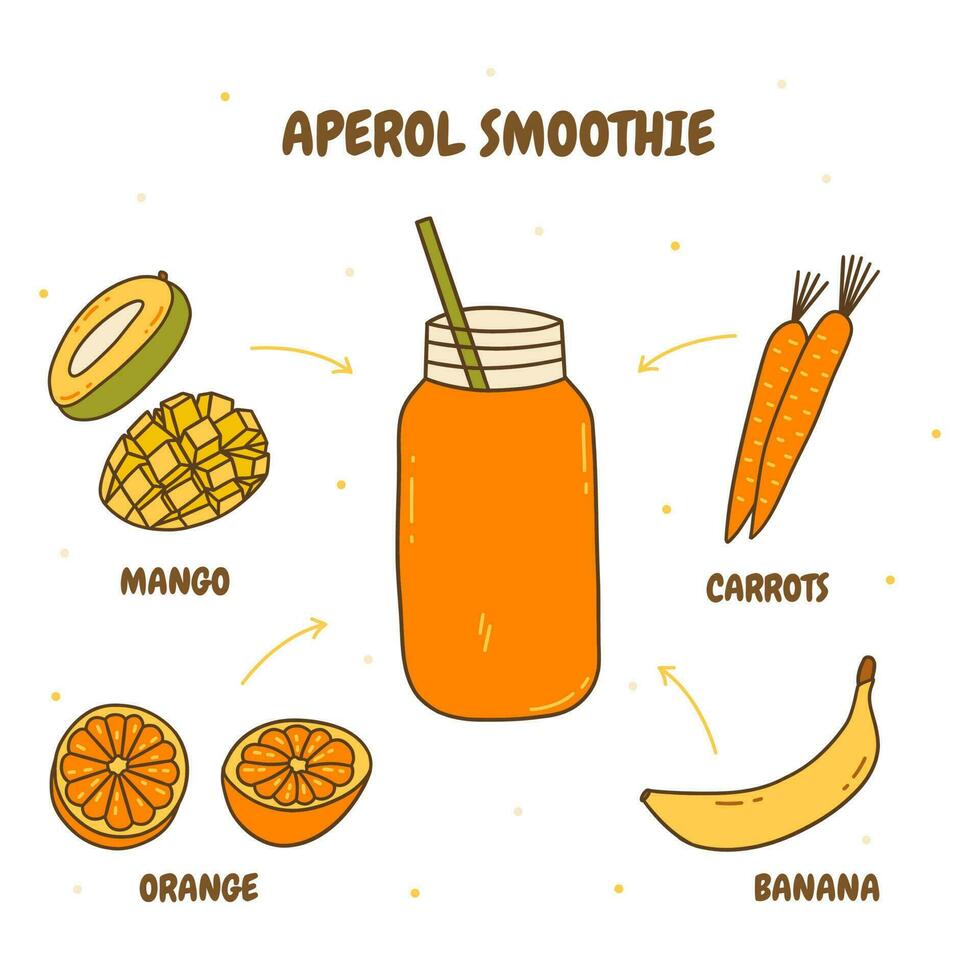This illustration features an Aperol Smoothie, prominently labeled in all caps across the top. The design is set against a white background. At the center of the image, a mason jar filled with an orange liquid sits with a beige top and a green straw. Surrounding the jar, there are detailed illustrations of the smoothie ingredients: two whole carrots, a single banana, two halves of an orange, and two mango halves—one with the pit exposed and the other sliced into cubes with the peel arching inward. Arrows point from each ingredient toward the jar, indicating they are the components of the Aperol Smoothie. Additionally, the backdrop contains subtle yellow dots, adding a playful touch to the diagram.